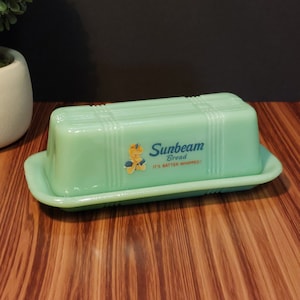The image showcases a glossy, mint-green ceramic butter dish resting on an artificial-looking, shiny wooden table. The butter dish, featuring the brand name "Sunbeam" and an old logo of a girl eating a slice of bread with butter, consists of a rectangular base with curved edges and a lid shaped like a stick of butter or a small bathtub. The background reveals a black-painted wall and a barely visible potted plant in the upper left corner, enhancing the focus on the butter dish as the central element of the composition.